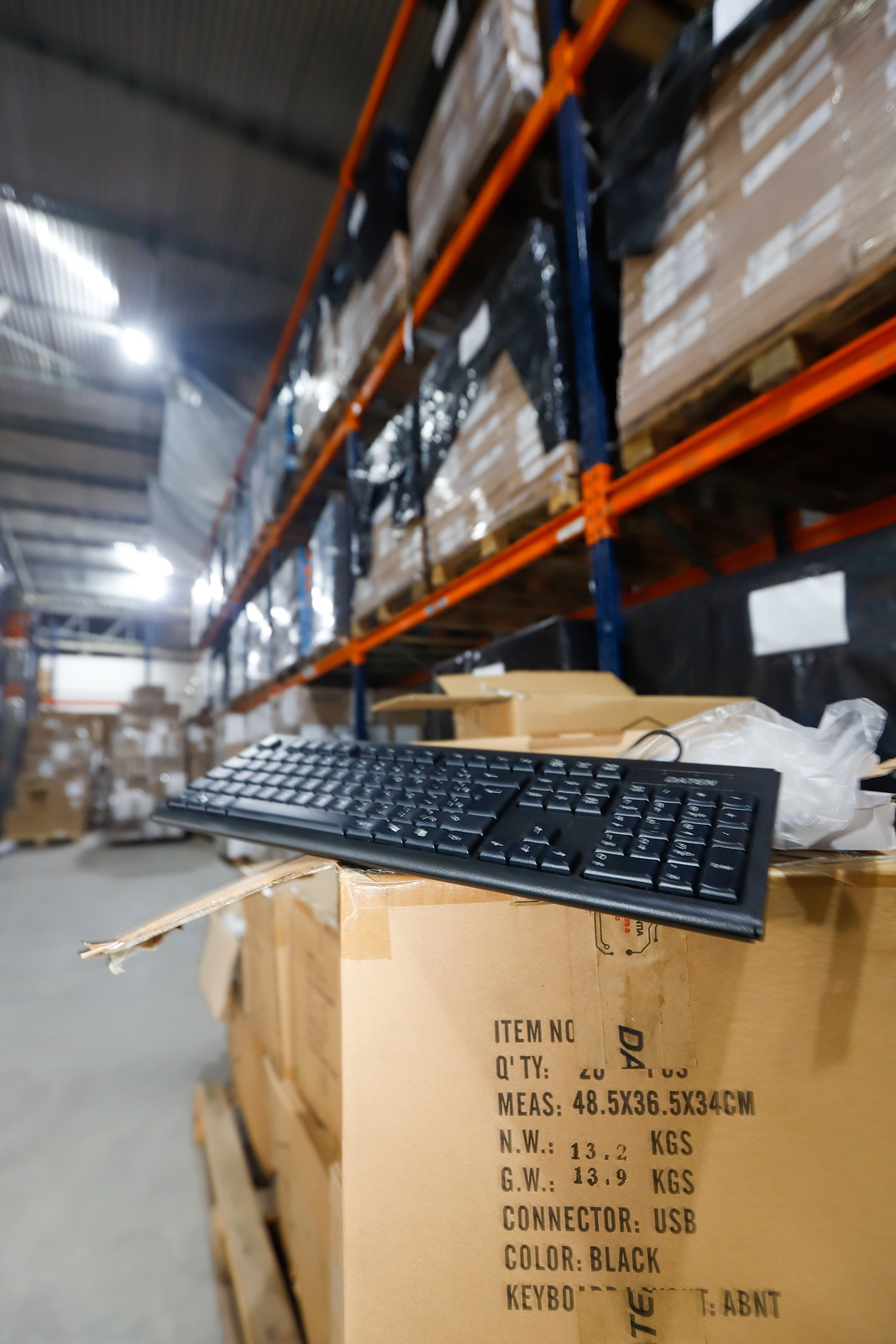The image depicts the interior of a bustling industrial warehouse or factory, characterized by its grey floor, and a background lined with orange shelving supported by blue brackets, stacked with blurred cardboard boxes of varying sizes. In the foreground sits a large open cardboard box, sealed with brown tape at the top and bottom, resting on a wooden pallet. On top of this box, there is a black keyboard and an empty, wadded-up clear plastic bag. The box displays various labels, including "item number," "quantity," "MEAS 48.5 x 36.5 x 34 cm," "N.W," "G.W," "connector USB," "color black," and "keyboard." The overall scene emanates a busy, industrial atmosphere akin to a Home Depot warehouse, filled with aisles and an array of boxed merchandise.